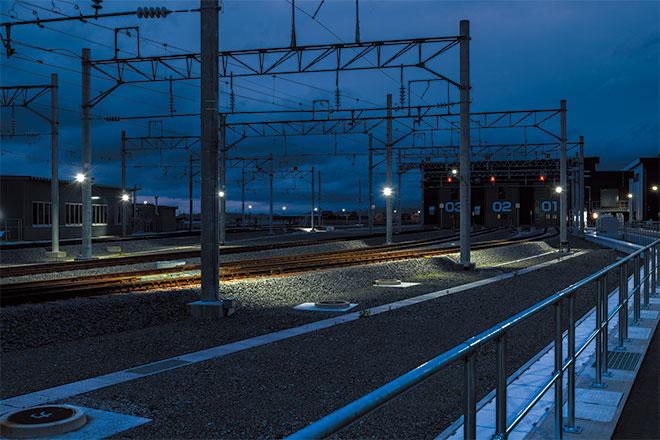This nighttime cityscape image captures the essence of a commuter rail station under a deep blue sky with slight variations of dark and light due to distant clouds or smoke. Dominating the scene are the tracks of the commuter train, bordered by an array of metal poles and electrical cables essential for the train's operation. Above the tracks, multiple thin black lines and crisscrossing cables create a complex network resembling a tall volleyball net, underscoring the functional but intricate infrastructure. On either side of the tracks, four identifiable poles stand in alignment, with additional poles dispersed randomly, further adding to the intricate web of lines.

In the distance, city lights glimmer, accompanied by smaller yellow and white dots lining the track, likely functioning as signal lights for train management. The right side of the image features a pedestrian waiting area bordered by a silver metal barrier, composed of vertical and horizontal thin silver poles, ensuring safety and organization. Noteworthy are three black structures visible in the distance, possibly toll booths or vehicles, each marked with numbers in blue – 03, 02, and 01 – standing out against the nuanced blue backdrop. The horizon's soft ombre effect blends from deep to lighter blue, accentuating the atmospheric depth of the scene while the light blue stripe and various grey and white spots add contrast and details to the overall composition.